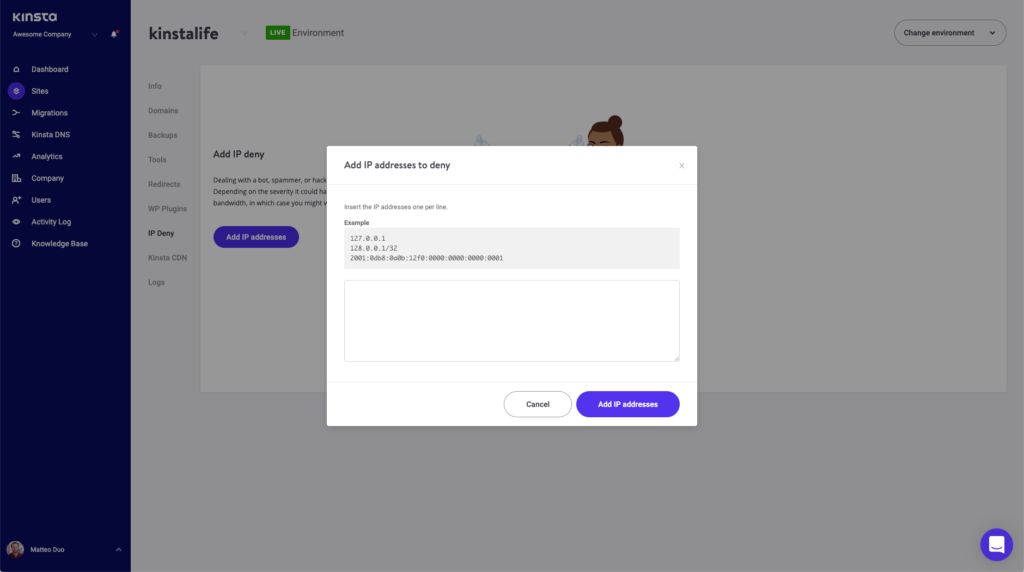The website interface for KNSTA’s Awesome Company features a vertical blue band on the left side with a series of navigation options: Dashboard, Sites, Migrations, KNSTA DNS, Analytics, Company, User, Activity Log, and Knowledge Base. Adjacent to this on the right, the main section of the page displays the 'KNSTA Live Environment' with a notice indicating 'Add IP Denied.' This area is overlaid with a translucent gray filter.

A prominent white pop-up window appears, titled 'Add IP Address to Deny.' The window prompts users to enter IP addresses, each on a separate line, providing examples such as '127.0.0.1/32' and '2001:0db8::/32'. The resolution of the pop-up obscures some of the text. It includes an empty data field for input, a 'Cancel' button, and a blue 'Add IP Addresses' button with white font.